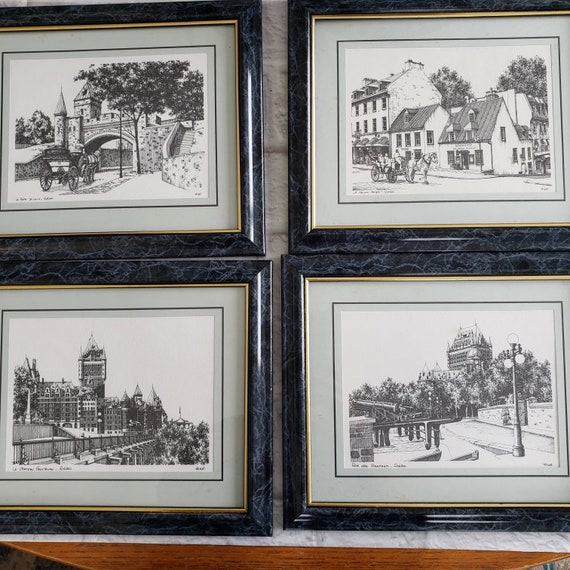This color photograph showcases four framed black-and-white illustrations arranged in a square pattern. The frames are dark blackish-brown with a glossy faux marble finish, featuring lighter gray veining meant to mimic stone, and a gilt gold lining on the inner edges. Each illustration is matted uniformly with a pale gray mat and a dark blue border, giving a double-matted appearance.

The illustrations depict various outdoor architectural scenes. 

1. **Top Left**: An intricate scene with a turret reminiscent of a medieval castle and an arched stone bridge. A horse-drawn wagon is poised to pass underneath the arched structure.
2. **Top Right**: An image of an old-fashioned inn with dormer windows and tall chimneys, flanked by shorter buildings and trees. Another horse-drawn carriage stands in front of the inn.
3. **Bottom Left**: A depiction of tall, elaborate brick buildings, possibly of English architecture, with towers and a terraced wall in the foreground.
4. **Bottom Right**: A street scene featuring a double lamppost with three globe lamps, a railing, and a stone fence pillar, leading to a tall building framed by rows of trees.

The detailed, pen-and-ink style drawings convey a timeless, historical ambiance.